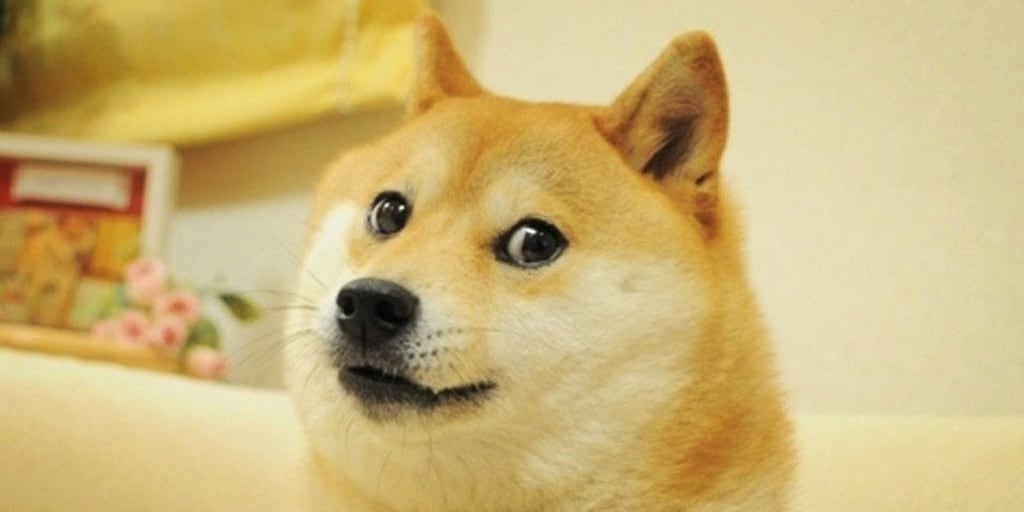This is an adorable and detailed close-up photo of a fluffy, golden-colored dog with white fur around its face, taken indoors. The dog, zoomed in on its face, has dark, expressive eyes that are looking towards the right, a nice-sized black nose, and black whiskers clearly visible where they sprout from the top of its slightly open mouth. The dog’s ears are sticking up with a hint of pink along the edges. Captured in what seems to be someone's home, possibly on a white sofa, the background features a white wall, a table behind the couch with pink roses, a framed picture, and a yellowish curtain hanging to the upper left. The charming setting and the delightful nature of the dog evoke the iconic image of the Doge meme.